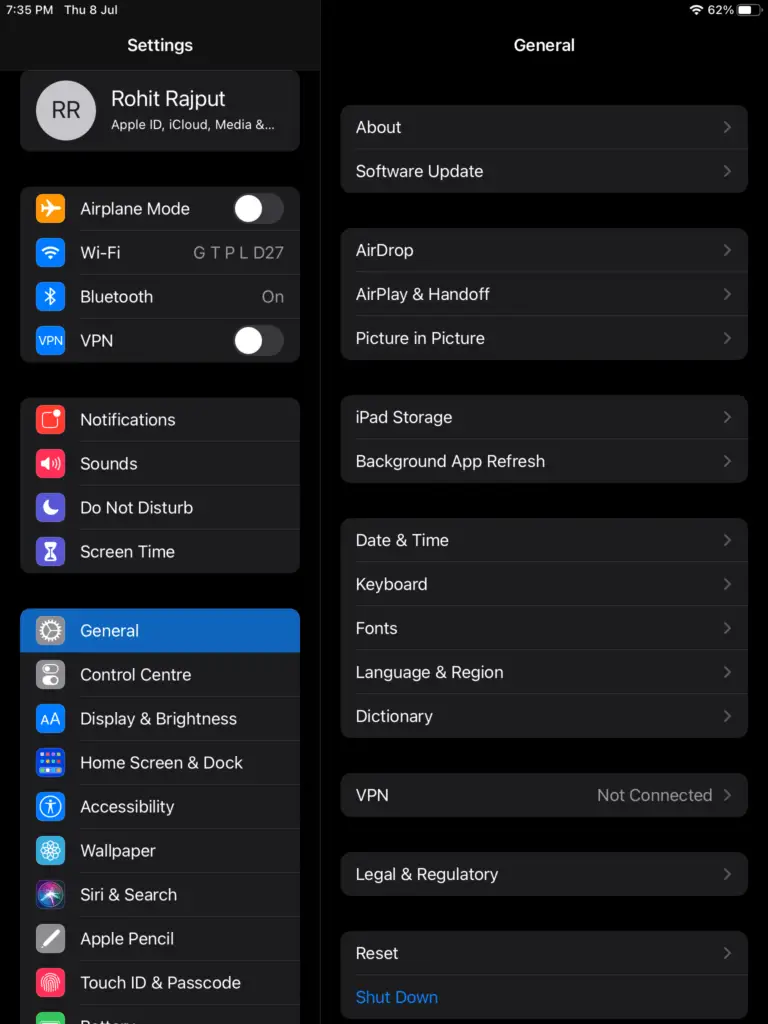Screenshot of an Apple Device in General Settings

This detailed screenshot showcases an Apple device's settings menu prominently displayed on a dark mode interface. On the far left, the main settings menu features the user’s name and a link to their Apple ID. Standard options such as Airplane Mode, Wi-Fi, Display, and Wallpaper settings are clearly visible. 

The user has navigated to the General settings section, revealing options like About, Software Update, iPad Storage, and Date & Time, among others. While none of these specific options are highlighted or selected, their presence is evident. 

Additional details include the device information displayed at the top of the screen – it is 7:35 PM on Thursday, July 8th. To the right, standard Apple indicators show the Wi-Fi connectivity symbol and the battery level at 62%. 

Overall, this screenshot provides a comprehensive view of the Apple device's interface and settings options.